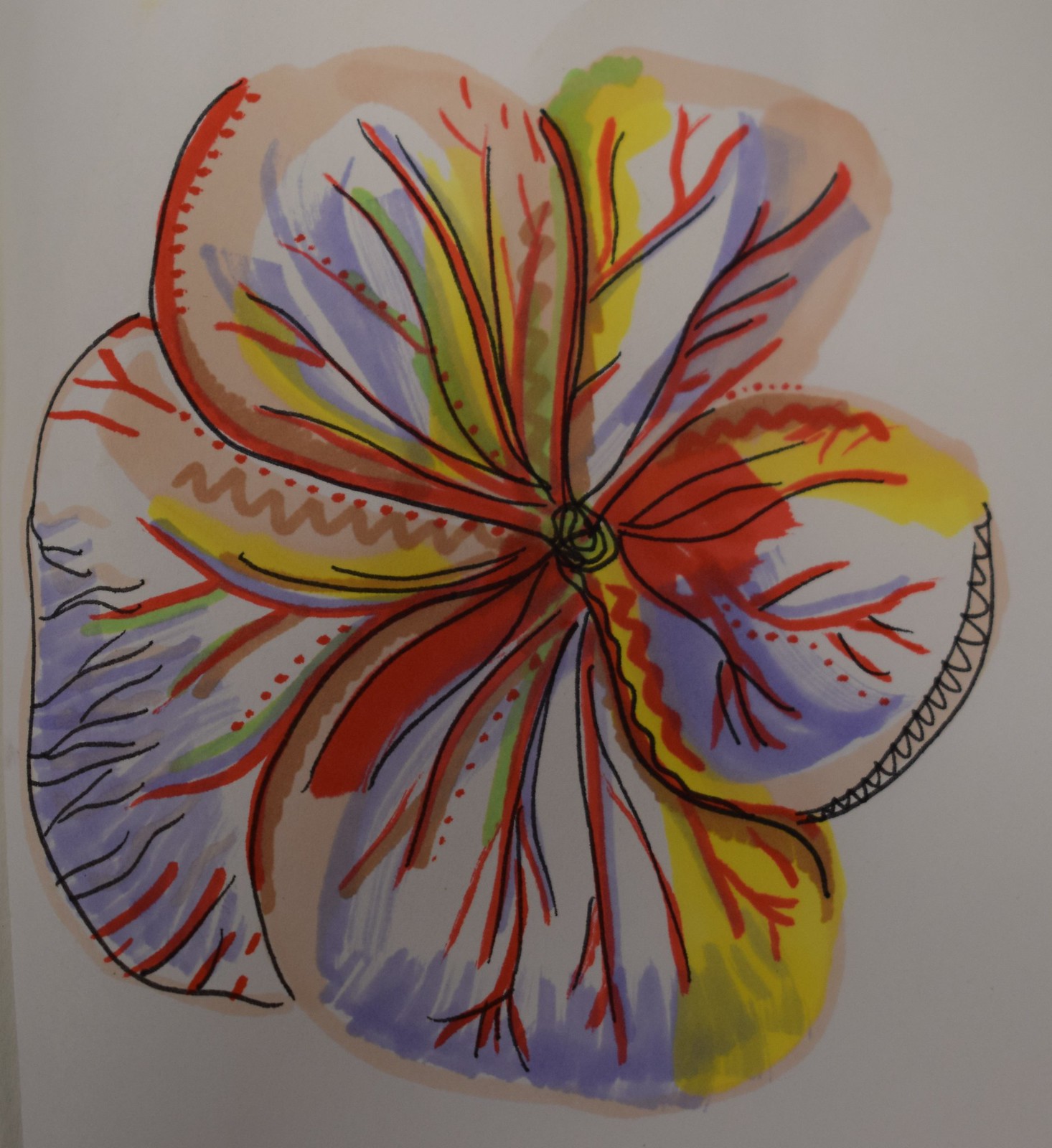This is a highly detailed close-up image of a flower set against a plain white piece of paper. The flower is the focal point of the picture, showcasing its intricate and unique features. Each petal displays its own distinct pattern and color scheme. The petal edges are lined with a vivid orange which fades towards the middle while remaining unlined towards the outer edges. 

One petal stands out with yellow and blue paint swipes in the background and a series of dots along its central vein. Adjacent to this, the next petal presents a gradient of colors, starting from yellow at the base, transitioning to white, and culminating in blue paint strokes. Another petal mirrors this pattern but adds a striking red circle at its lower end. 

A large petal with a blend of yellow, various shades of blue, and tan appears next. The tan sections fill the gaps not covered by other colors, adding depth to the flower. Behind all these petals, there is an overarching large petal adorned with black veins extending from the top and orange veins originating from the bottom. These orange veins are highlighted with an assortment of colors such as green, brown, blue, and yellow. Additionally, a brown zigzag pattern ascends next to a line of dots, further enriching the visual complexity of the flower.